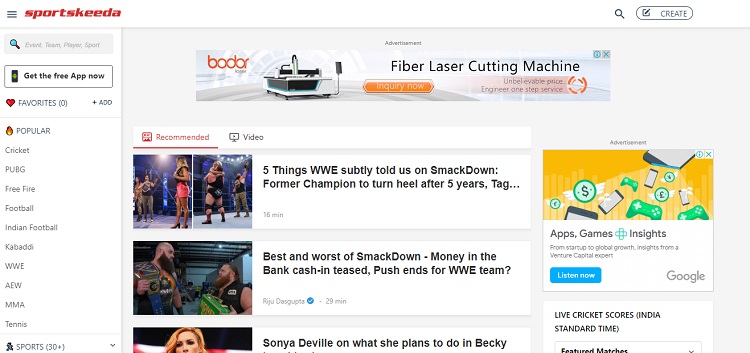Screenshot featuring a webpage with a predominantly white background. In the upper left corner, the company name "Sportskeeda" is displayed in bold red block text. To the left of the company name, there is a three-line menu icon.

Centrally positioned below is an image depicting a fiber laser cutting machine. In the upper left corner of this image, the brand name "Bodar" is written in yellow text. 

To the right of the machine image, an orange action button labeled "Inquire Now" is prominently featured. Adjacent to the button, the text "Unbelievable Price, Engineer One Step Service" is displayed, emphasizing the product's affordability and expert service.

In the lower right corner of the screenshot, there is a rectangular ad with a background gradient of yellow and orange. The ad is framed with the label "ADVERTISEMENT" at the top. Within the ad, there are illustrations of handheld games and cell phones. Below these illustrations, text in a white box reads, "Apps, Games, Insights from Startup to Global Growth, Insights from a Venture Capital Expert." At the bottom, a blue action box with the text "Listen Now" invites users to engage further.